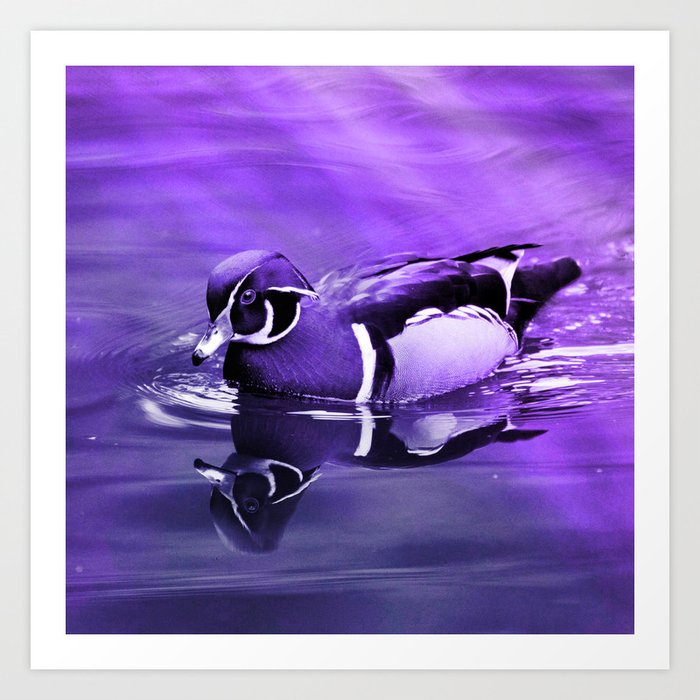The artwork, framed in white and hanging on a wall, features a striking image of a duck swimming in water, all rendered in shades of purple and dark blue. The entire scene is enveloped in a heavy purple hue, including the background and the water. The duck, identifiable as a mallard by its markings but not by its usual colors, has a predominantly dark purple head and body with a pointy beak that transitions from purple to white, ending in a black tip. The duck's underbelly and sides show a lighter purple or lavender hue with white stripes. You can see the duck's reflection in the water, and there are noticeable ripples and streaks of sunlight filtering through, casting lavender sunbeams onto the scene below. Despite the unnatural color palette, the duck appears to be actively swimming, with water breaking behind him, adding a dynamic element to the surreal and beautiful composition.